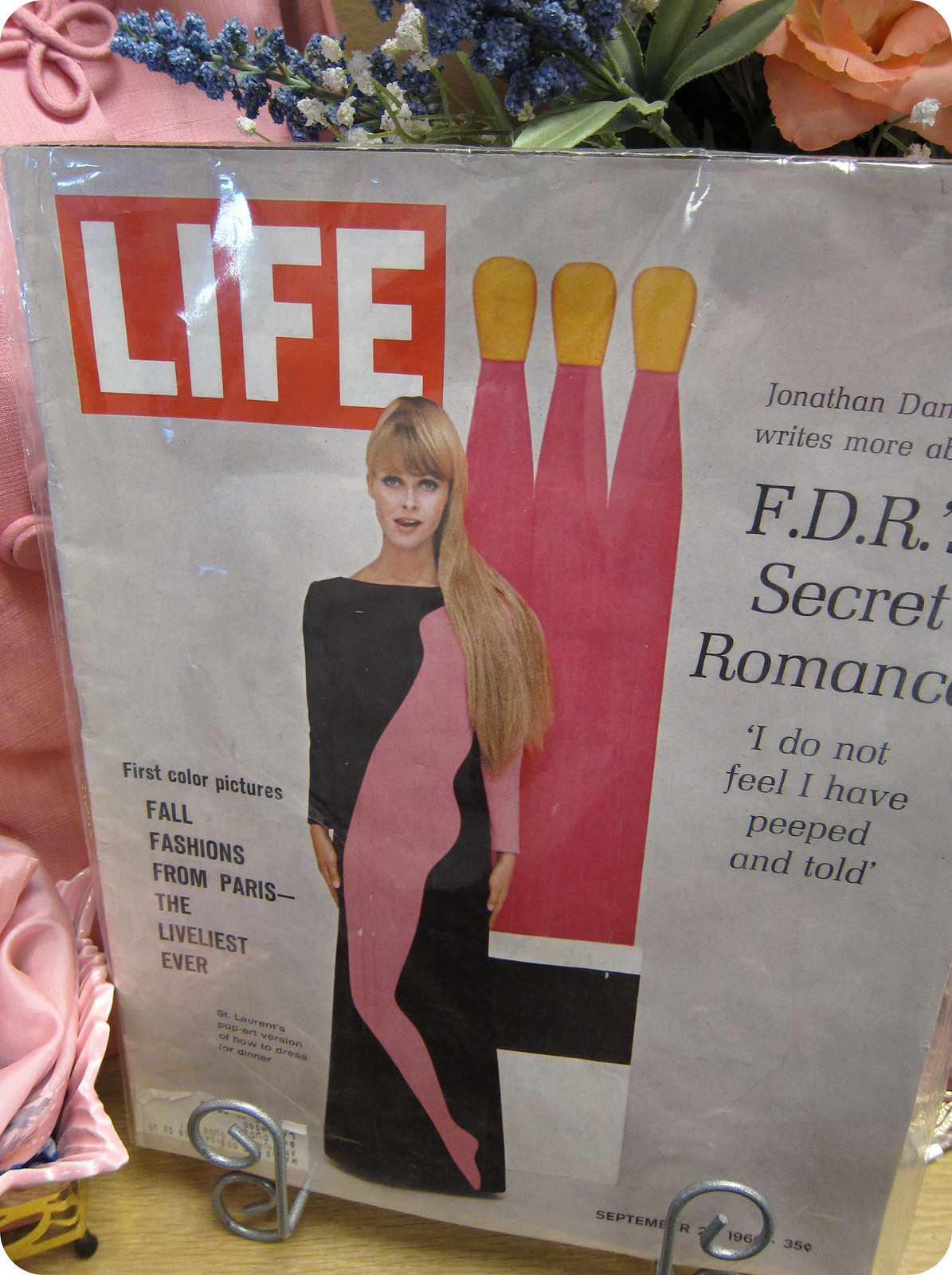This detailed illustration depicts a vintage Life magazine placed upright on a small silver stand that is positioned on a light beige wooden surface. Dominating the image, the magazine's cover features a woman with long blonde hair and bangs, adorned in a striking dress that is predominantly black with one pink sleeve and a silhouette pattern of a woman's body cascading down it. The cover announces bold headlines, including "Life First Color Pictures: Fall Fashions from Paris, the Liveliest Ever," and a tantalizing story about "FDR’s Secret Romance" accompanied by the intriguing subtitle, "I Do Not Feel I Have Peeped and Told." The magazine's signature red rectangle with the word "Life" in white letters is prominently displayed in the top left corner. Surrounding the magazine, there's a pink fabric pillow to the left and vibrant flowers in orange and blue hues can be seen in the background toward the top.